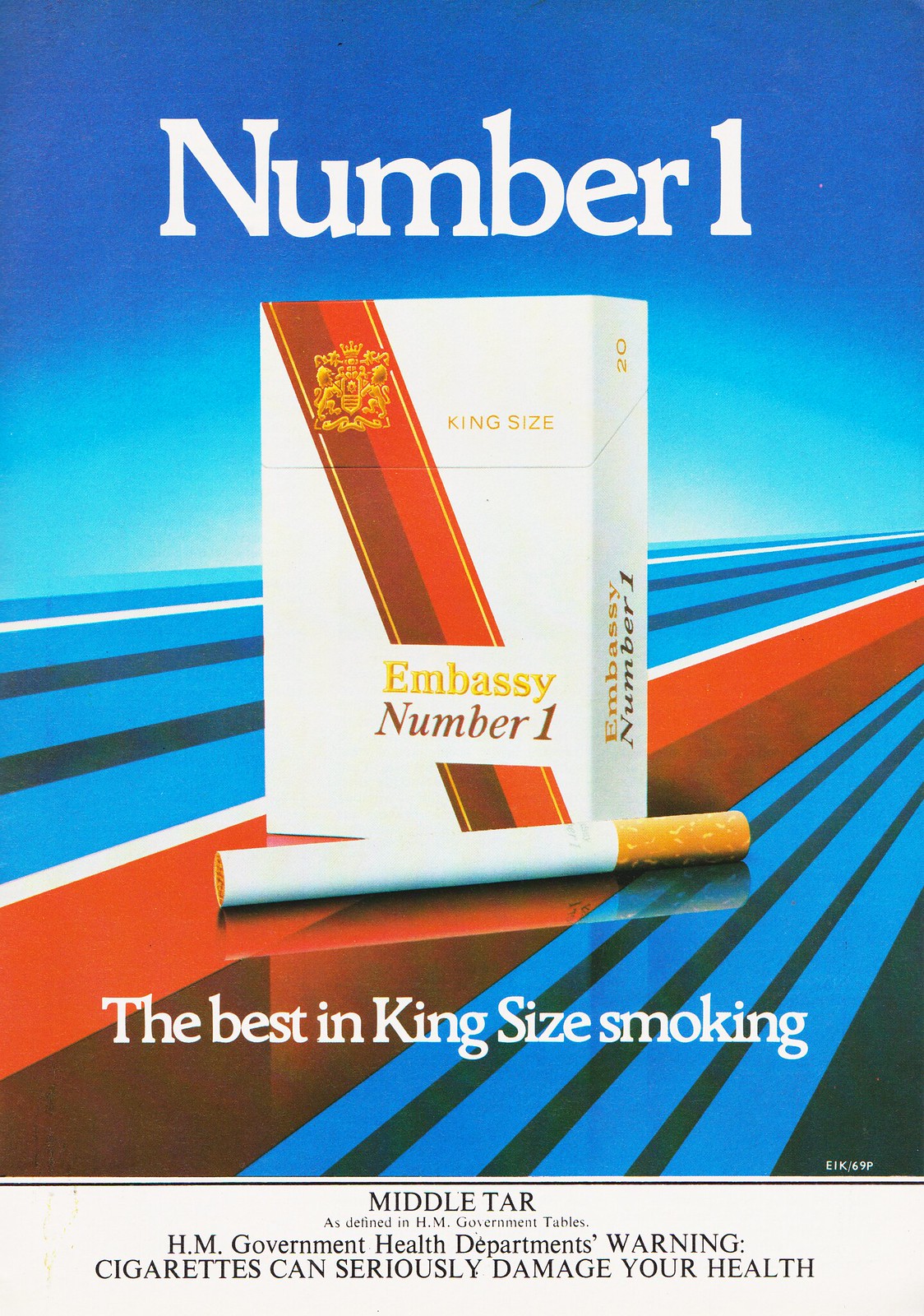The image is an advertisement for Embassy No. 1 cigarettes, depicted within a vertical rectangular box. At the top of the image, "NUMBER ONE" is prominently displayed in white serif lettering. Below this title, a white cigarette pack is showcased, adorned with a diagonal red stripe transitioning from a maroon hue at the bottom to a brighter red at the top. The pack features gold markings, including the word "Embassy" in gold and the designation "king size" at the top, along with the number "1" in red. A cigarette with a brown filter is placed horizontally in front of the pack. The background of the image consists of intersecting blue, white, red, and gray stripes that start from the bottom left and extend to the middle on the right. At the bottom of the image, the text "THE BEST IN KING SIZE SMOKING" is inscribed in white. Beneath this rectangular image, there is additional information stating "MIDDLE TAR," followed by a government health warning in Times New Roman font, declaring "CIGARETTES CAN SERIOUSLY DAMAGE YOUR HEALTH".